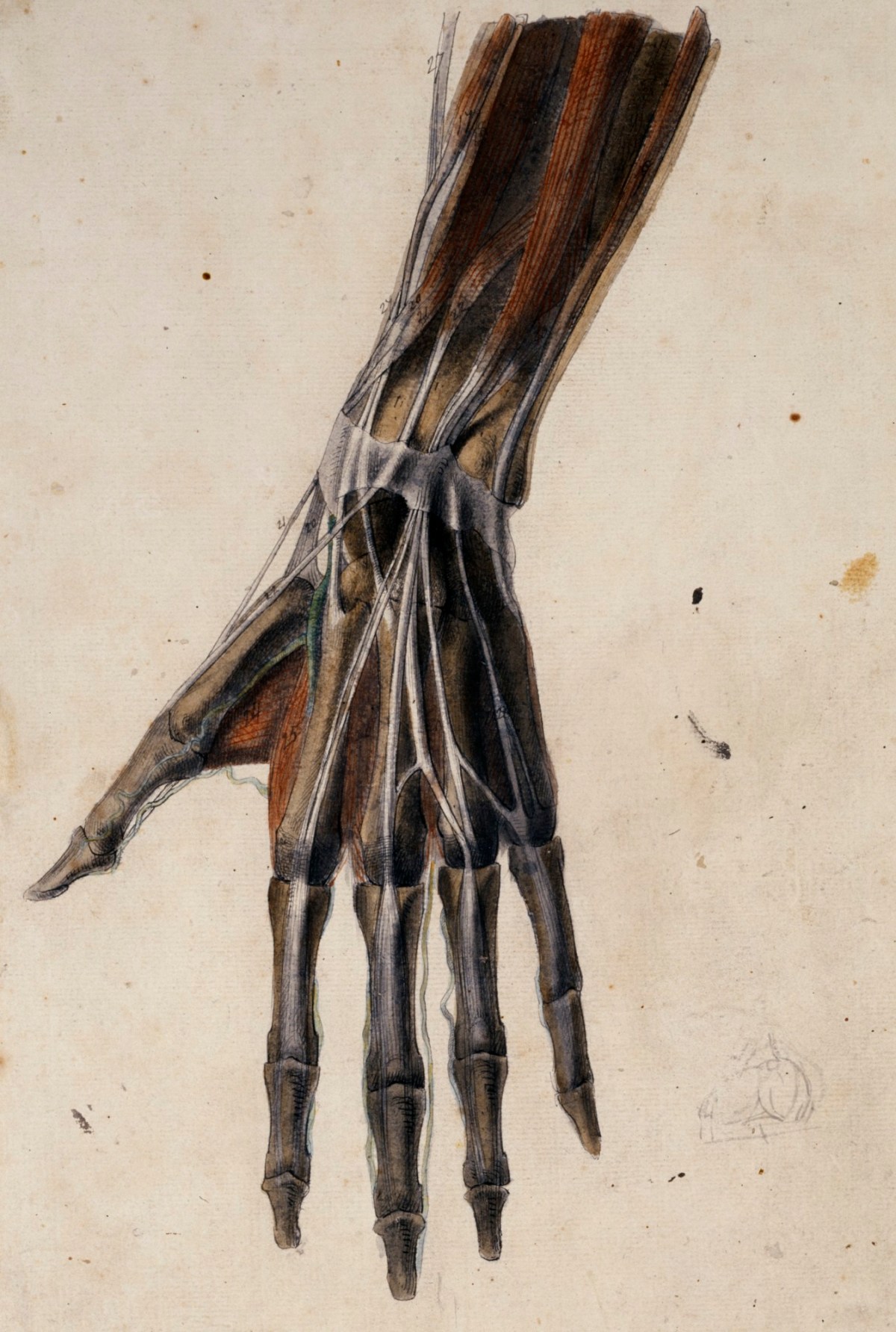The image portrays a detailed anatomical painting of a left human hand, descending from the top across a beige background. The hand lies flat with fingers and thumb spread, revealing an intricate view of the muscular, skeletal, and vascular structures inside. The muscles, rendered in dark red and brown hues, contrast with the bones depicted in white and gray. The tendons and thin bone-like structures are visible, extending from the hand's wrist through the fingers. The hand also shows detailed interconnections of veins and arteries, with a distinct webbing between the thumb and index finger. Additionally, black dots scattered across the image and a brown smudge add to its intricate detail.